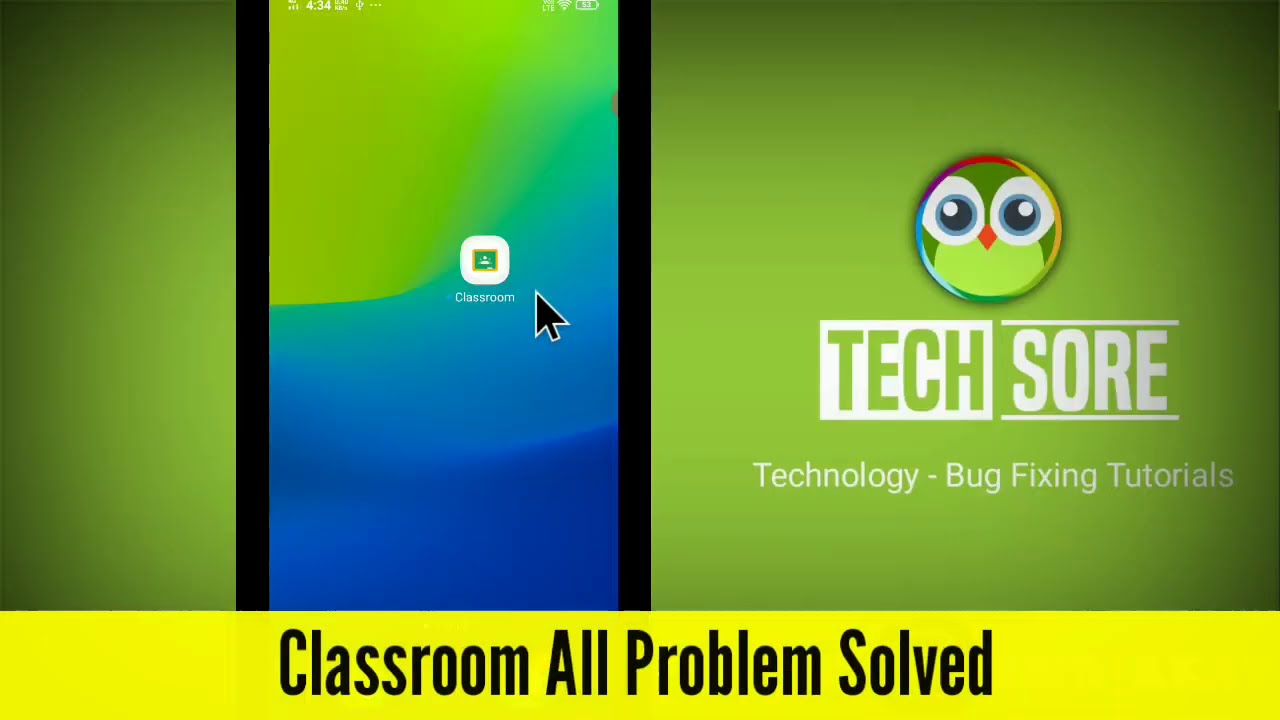The advertisement image for TechSor features a distinctive and vibrant design. Dominating the right side is an illustration of a small, cute, round bird in a simple yet playful style, acting as the logo for TechSor. The word "TechSor" is prominently displayed in white text against this logo, with the "Tech" part highlighted by a white background, making it stand out.

The entire background of the image showcases a green gradient that subtly transitions into black toward the center. Off to the left, there appears to be a partial view of a tablet or phone screen. The screen is cropped such that only the indicators for battery and WiFi are visible at the top, suggesting a mobile interface. This screen also features a single icon that reads "classroom," hinting at a potential app or portal related to their product.

Towards the bottom of the image, a yellow banner with centered black text declares, "classroom all problems solved," providing a clear message of the product's utility. The image's segmented layout and the vibrant colors contribute to its eye-catching and modern appeal, while the simple, yet effective design elements emphasize TechSor's focus on technology and problem-solving tutorials.